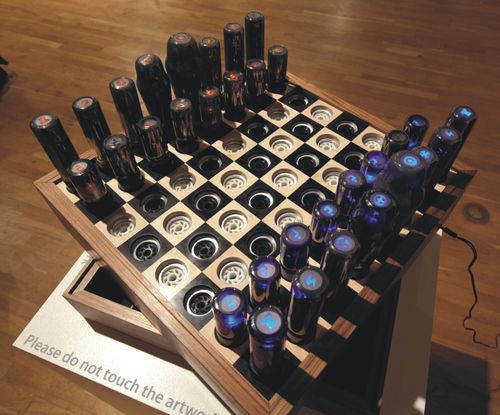This photograph captures an art installation designed to resemble a chess set, prominently displayed on a light brown wooden floor in a museum setting. The chess set rests on a pedestal featuring a sign with the words "Please do not touch the artwork" printed in black letters, emphasizing its artistic nature rather than its function as a traditional game board. 

The chess board itself is intricately crafted, featuring a checkerboard pattern with alternating black and beige squares and framed by a wooden edge. Below the board top, a wooden compartment stores the pieces. Each set of pieces is highly abstract and exudes a metallic, futuristic aesthetic. The pieces are split into two opposing sides: one side is adorned with blue lights at the tips, while the other side features red lights. Both sets of pieces are meticulously lined up, ready for a game, with the blue-lit pieces distinctively illuminated in the photograph.

The entire setup is enhanced by the inclusion of electronic elements, with wires and components integrated seamlessly into the design, giving the sense that the pieces light up possibly through interaction or movement. This captivating blend of traditional chess motifs with modern, electronic elements underscores the innovative nature of the artwork.